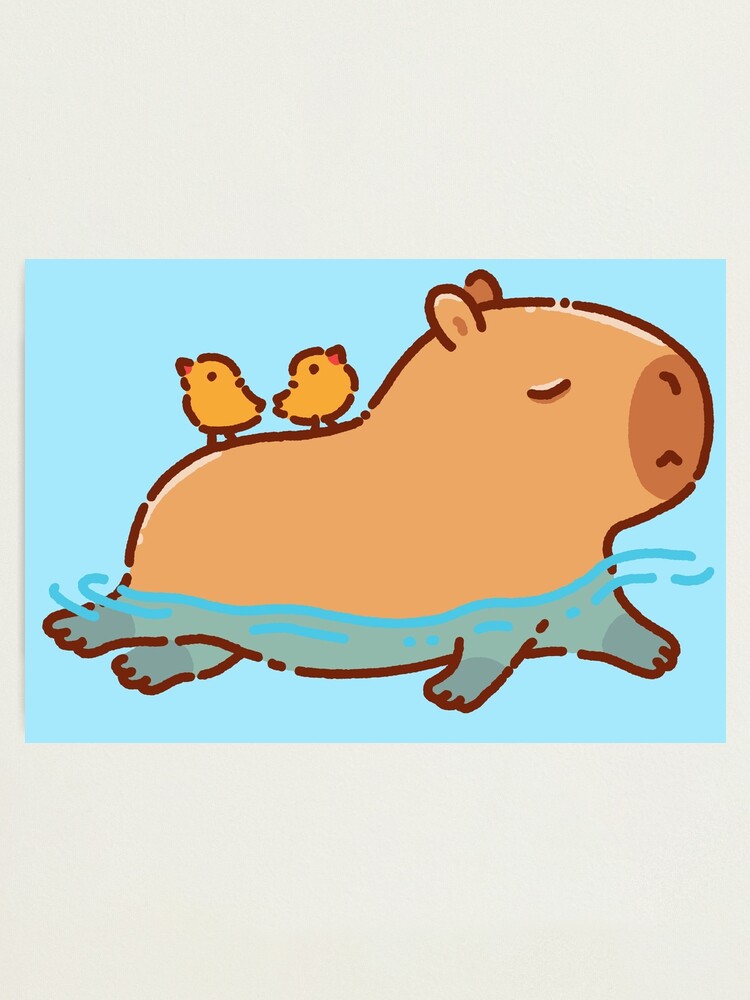This is a simple cartoon drawing on a gray piece of paper featuring an orange-peach colored animal that appears to be either a miniature pig or a hippopotamus, outlined in dark brown. The creature is situated in the center of a light blue square, surrounded by blue lines that indicate it is swimming. The animal has four little legs and its belly submerged in the water, while its snout, which is a lighter brown color, and two round ears are above the surface. Its single visible eye is closed, giving it a look of blissful peace. Perched on its back are two small yellow-brown birds about the size of finches, with dark beady eyes and little red or orange beaks. One bird is facing left and the other facing right. The background is off-white, complementing the serene and whimsical nature of the scene.